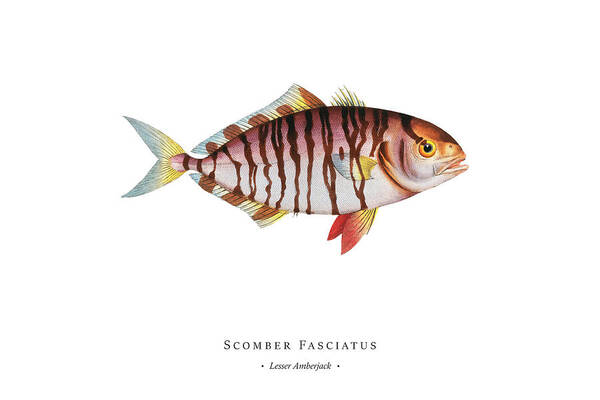This highly detailed illustration depicts a fish, specifically identified at the bottom of the image with the text "Scomber fasciatus" and "Scomber fasciatus in italics, Lesser Amberjack" flanked by dots on either side of the latter name. The fish is illustrated with exquisite precision, evoking the delicate strokes and nuanced color that suggest the use of colored pencils. 

The fish is oriented facing to the right, revealing its large, yellow eye with a prominent black pupil and a slightly open mouth. Two reddish-yellow fins emerge from the underside of the fish, complemented by two elongated fins towards the rear, adorned with alternating brown stripes. The tail, featuring a distinctive two-pronged shape, starts with a yellow base and transitions to blue tips.

The body of the fish exhibits a gradation of hues: pinkish tones dominate the upper part while the belly transitions to a lighter, whitish shade. Additionally, the gills are tinted with subtle orange or brown undertones, and several brownish stripes run along the length of the body, adding to the rich detailing of the illustration. The backdrop is a uniform shade of white, which allows the vibrant colors and intricate details of the fish to stand out prominently.